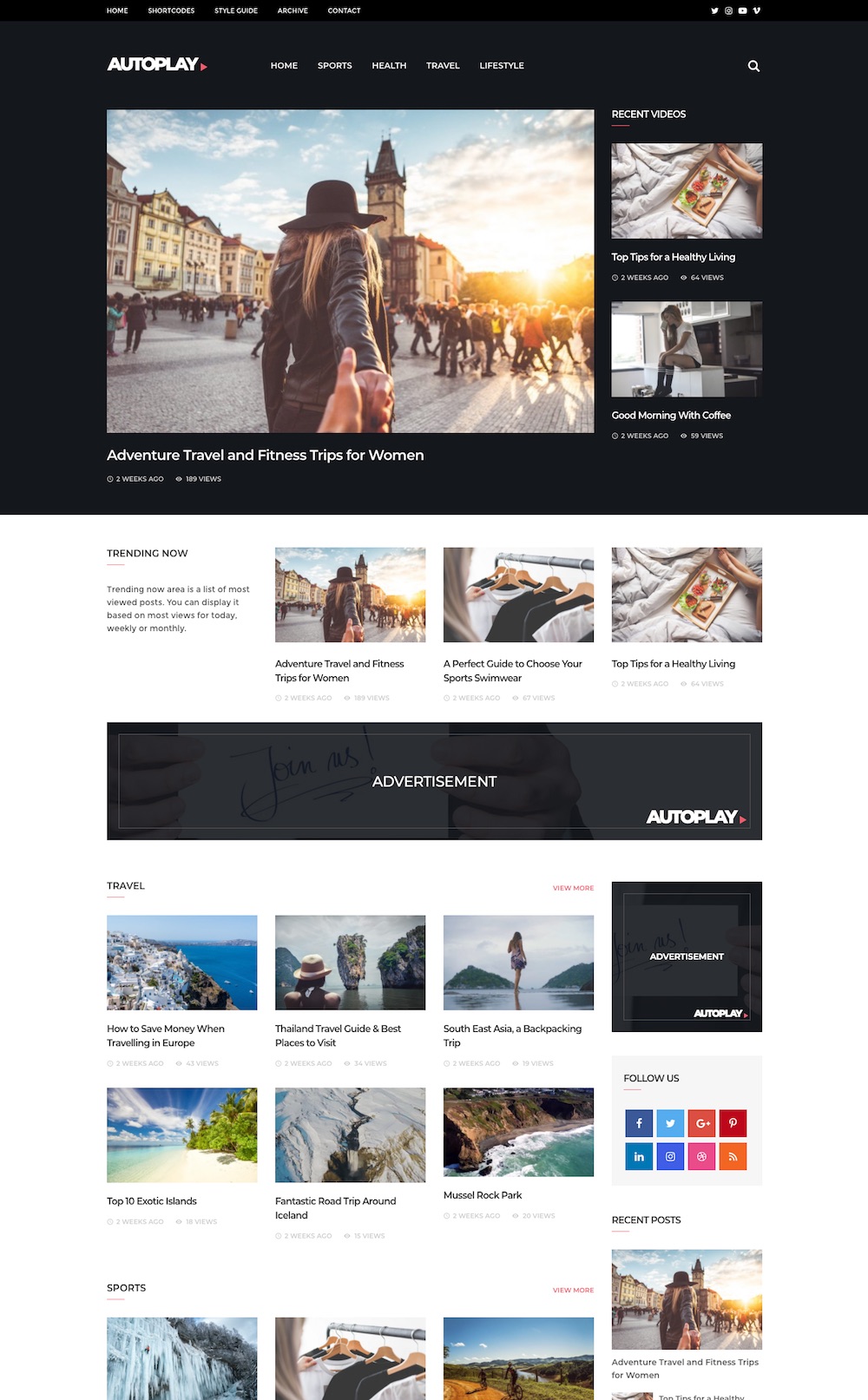A screenshot of a vibrant, user-friendly website dedicated to women's interests and travel. The homepage features a navigation bar offering categories such as "Sports," "Health," "Travel," and "Lifestyle." Prominently displayed is an image of a stylish woman in a hat, exploring a picturesque European town, possibly in a historical square with cobblestone streets. This image encapsulates the theme of travel and adventure. Below, the website hosts a collection of articles providing travel tips and lifestyle advice, alongside various embedded links. An autoplay advertisement is present, followed by a series of thumbnail images linking to additional articles, both within the site and externally. These thumbnails highlight enticing travel destinations like exotic islands and Southeast Asia, enriching the user’s experience by offering a diverse array of travel-related content and suggestions.